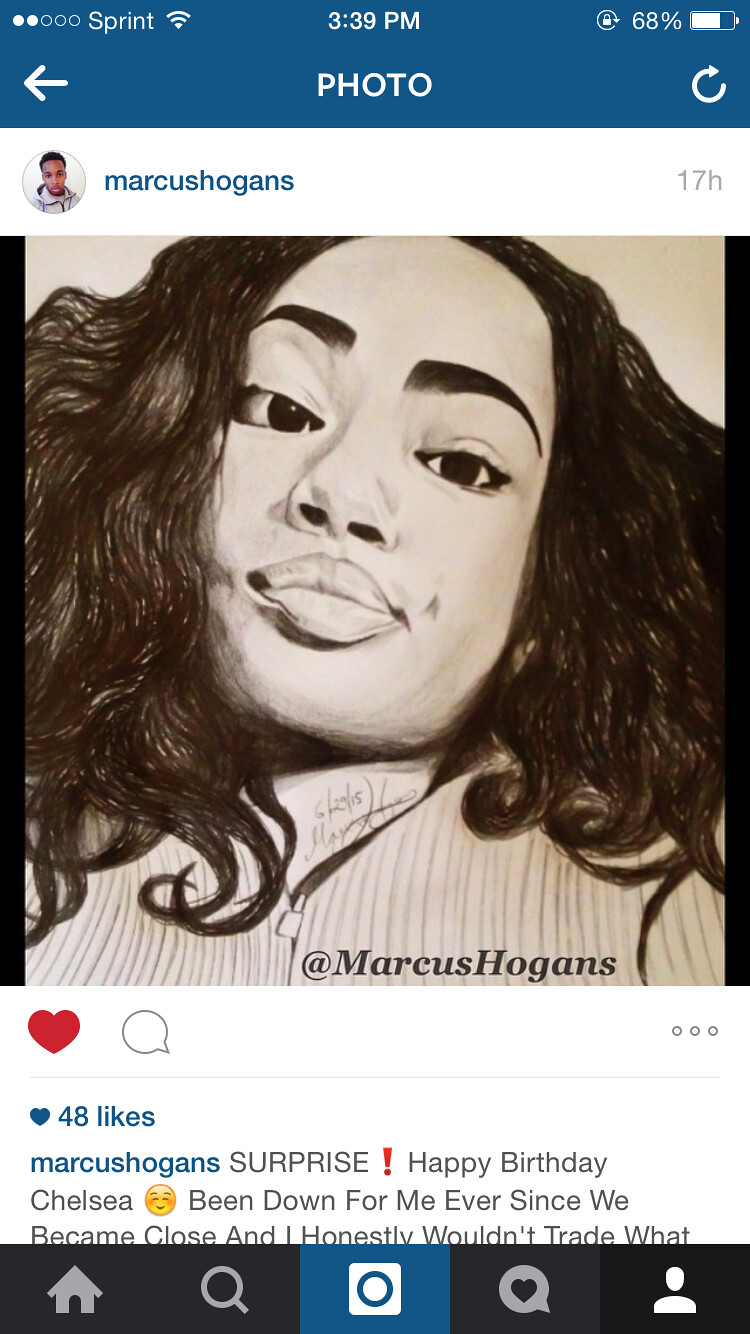In this image, we see a black and white style sketch against a light pink background, likely captured from a website or cell phone screen resembling social media. 

At the top, the interface displays “Sprint” as the network provider, and the timestamp reads 3.39 PM. The battery indicator shows 68% remaining. A dark turquoise bar at the top features the word "photo" in white letters. On the screen, a white arrow pointing left and a refresh symbol are visible.

Prominently featured is an image of a woman with dark, curly hair falling to her shoulders, lightly dark skin, and large, closed lips. Her eyes and eyebrows are also dark. She is dressed in a lightly gray, vertically striped blouse with white lines between the stripes, or possibly a striped zippered jacket.

The username "Marcus Hogan's" is displayed in black lettering above, with “17H” to indicate the time since posting. Below, a message reads: "Surprise! Happy birthday Chelsea, been down for me ever since we became close and I honestly wouldn't trade what…"

At the bottom of the image, we see a blue heart icon indicating 48 likes, along with a red heart and a little text box. Various other symbols are present, including a home symbol suggesting navigation options on the site.